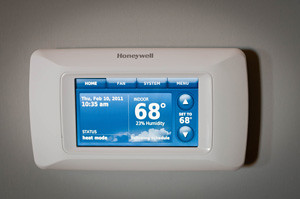The image depicts a small, rectangular digital thermostat mounted on a gray wall. The background has a subtle interplay of shadows and light, creating a sense of depth and dimension despite its otherwise smooth surface. The corners of the gray wall are darker, gradually transitioning to a lighter gray near the center due to a central light source, which highlights a shadow cast by the thermostat itself.

The thermostat, bearing the Honeywell brand in gray letters, has a modern design with white, rounded edges. Its surface is slightly protruding, adding to its three-dimensional appearance. The device features a digital display with a gradient blue background, showing the current temperature, date, and time. Below the display, there are up and down arrows, presumably for adjusting the settings. This precise lighting and detailed thermostat design create a focus point against the nuanced gray backdrop.